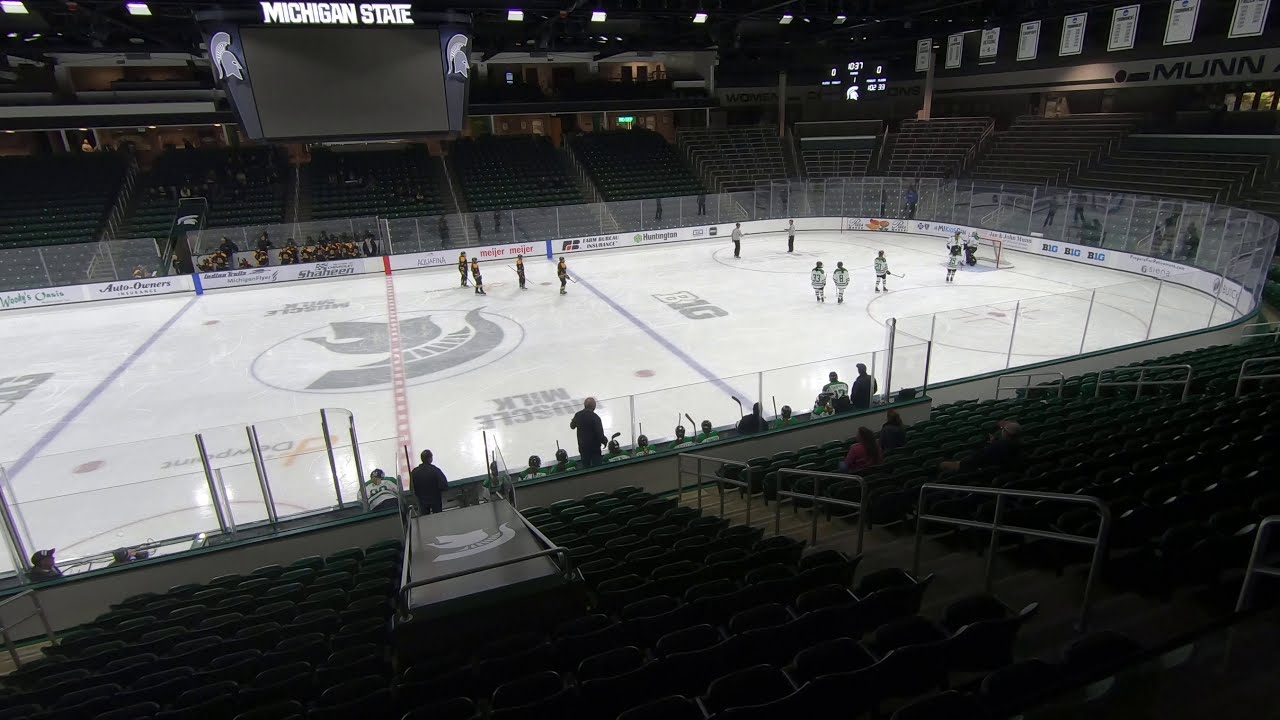This detailed photograph captures an indoor ice hockey stadium from the stands, showcasing not only the ice rink but also the surrounding seating areas. The ice surface is primarily white, adorned with various patterns including a prominent "B1G" and the word "Milk." At the center of the rink, a large image of a traditional warrior helmet stands out. The black chairs in the stands host spectators, adding to the vibrant atmosphere of the large, multi-tiered building. On the ice, players from two distinct teams are competing: one team in white jerseys and the other in jerseys that are mainly black with yellow and red details. Additional players and coaches are visible on the sidelines, contributing to the dynamic scene. Suspended from the ceiling is a display screen bearing the words "Michigan State" in white letters, providing a focal point above the action.